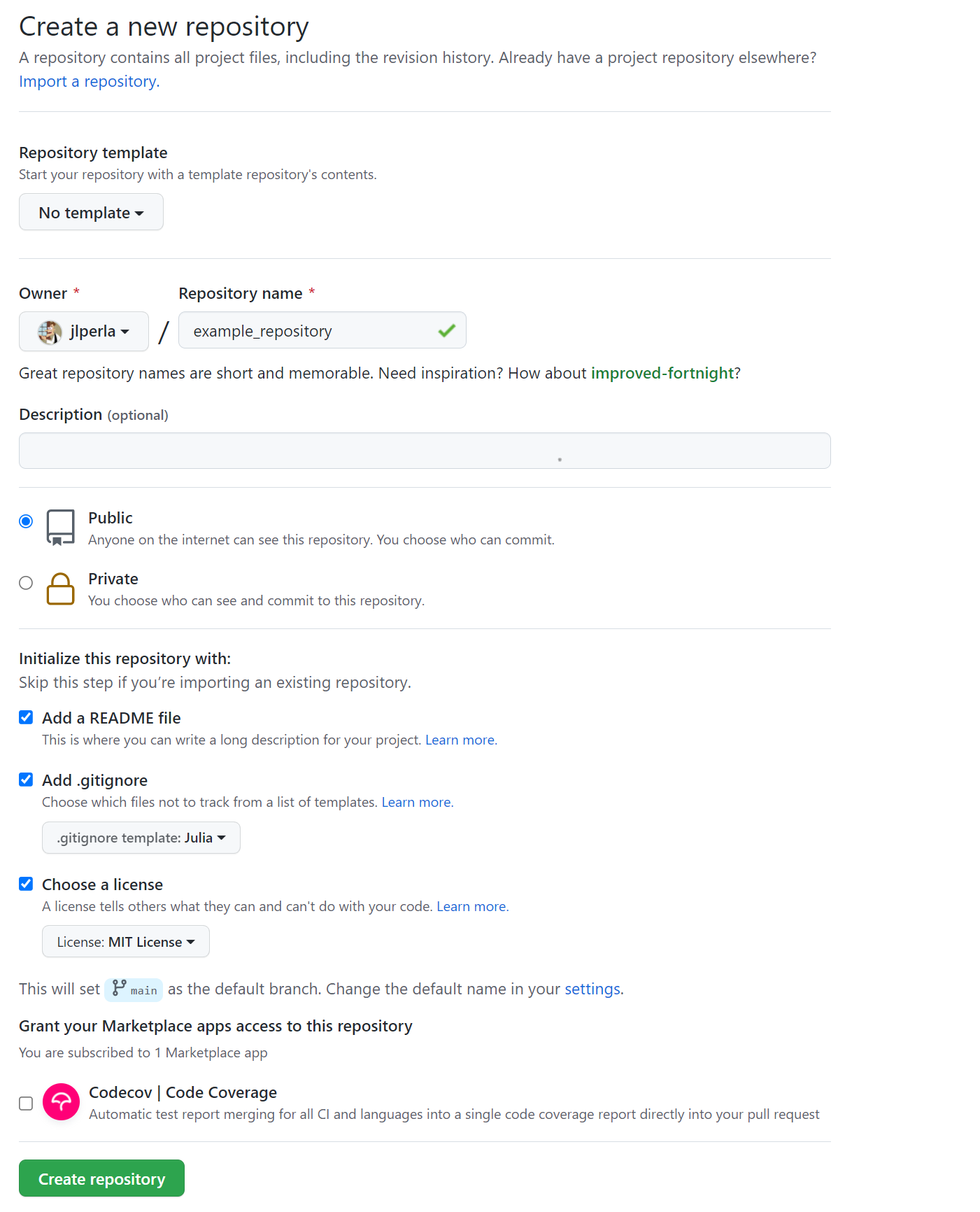The image shows a form for creating a new repository with the following details:

At the top, against a white background, there is a black header text that reads: "Create a repository. A repository stores all project files, including the revision history. Already have a project repository elsewhere?"

Below this header, there is a blue link that states: "Import a repository."

A thin gray line divides the sections, followed by the label "Repository template" in black text. The section explains: "Start your repository with a template." Inside a gray box, it says "No template" in black text.

Another thin gray line separates this from the next section, where in black text, it says "Owner" with an asterisk (symbolizing a required field) next to it. Below this, it says "Repository name" followed by a red asterisk, indicating the name is also required. There is a box with two fields: the first field shows "J-L-P-E-R-L-A" followed by a slash, and the second field contains "example-repository" along with a green check mark indicating approval.

Below this, black text reads: "Great repository names are short and memorable. Need inspiration? How about 'Improve-for-you'?" with "Improve-for-you" in green text.

Next, the label "Description (optional)" appears in black text, followed by a long, gray rectangular box for input.

Another thin gray line follows this, and beneath it, there are options for the repository's visibility: 

- "Public: Anyone on the internet can see this repository. You can choose who can commit."
- "Private: You can choose who can see and commit to this repository."

Next to these options, there are two circles for selection, with the "Public" option selected and highlighted in blue.

Another thin gray line separates the final section, which says: "Initialize this repository with:" This section advises to skip the step if importing an existing repository, and includes options to:

- "Add a README file"
- "Add a .gitignore"
- "Choose a license"

These options are provided to help properly set up the new repository.